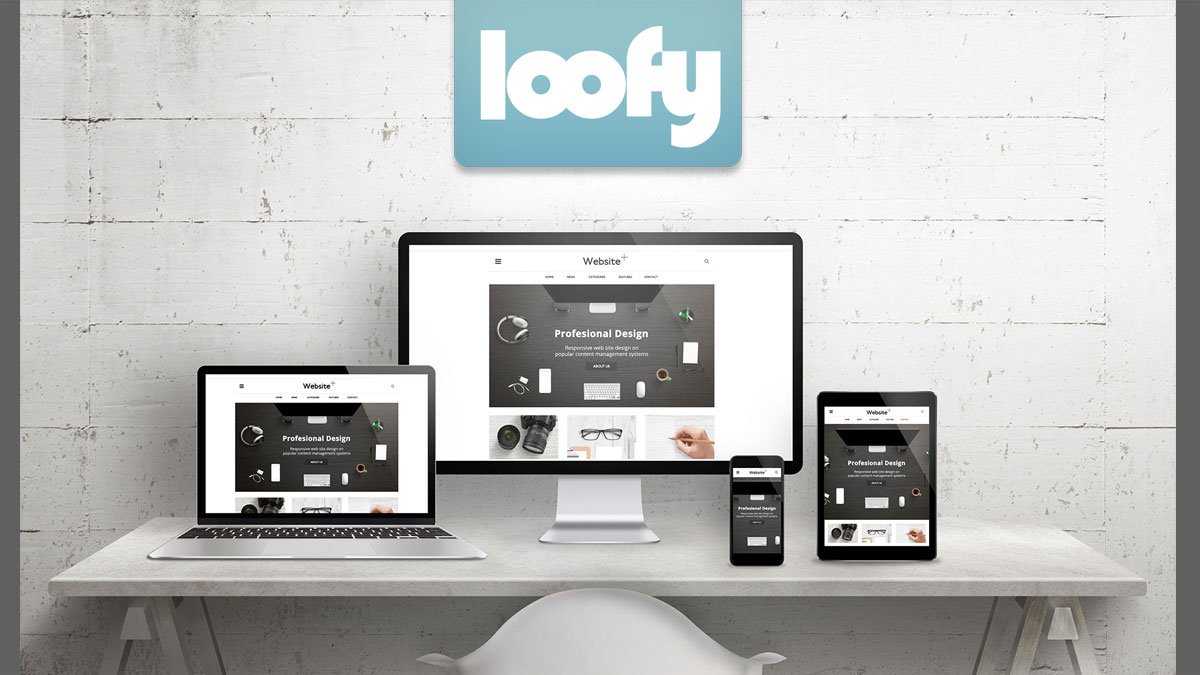The image appears to be an advertisement set against a white wall that shows signs of wear, with peeling paint giving it a dingy, run-down appearance. Along the side are two black vertical bars. Central to the scene is a grayish-teal sign with the playful, jaunty font in white spelling out "Luffy."

Below the sign is an off-white, slightly gray-toned desk, cluttered with multiple electronic devices. A silver laptop with a black keyboard displays a sample website titled "Black Website," highlighting professional design with an image of a workspace featuring earphones, a keyboard, a cup of coffee, some paper, and a green object. Next to the laptop is a desktop monitor with a thin black bezel and a silver stand, also showing the same workspace image but with additional details, including a black camera, black glasses, and a light-skinned hand holding a pencil.

Additionally, there is a cell phone and a tablet on the desk, each mirroring the same website. A white chair is positioned in front of the desk, completing the scene.